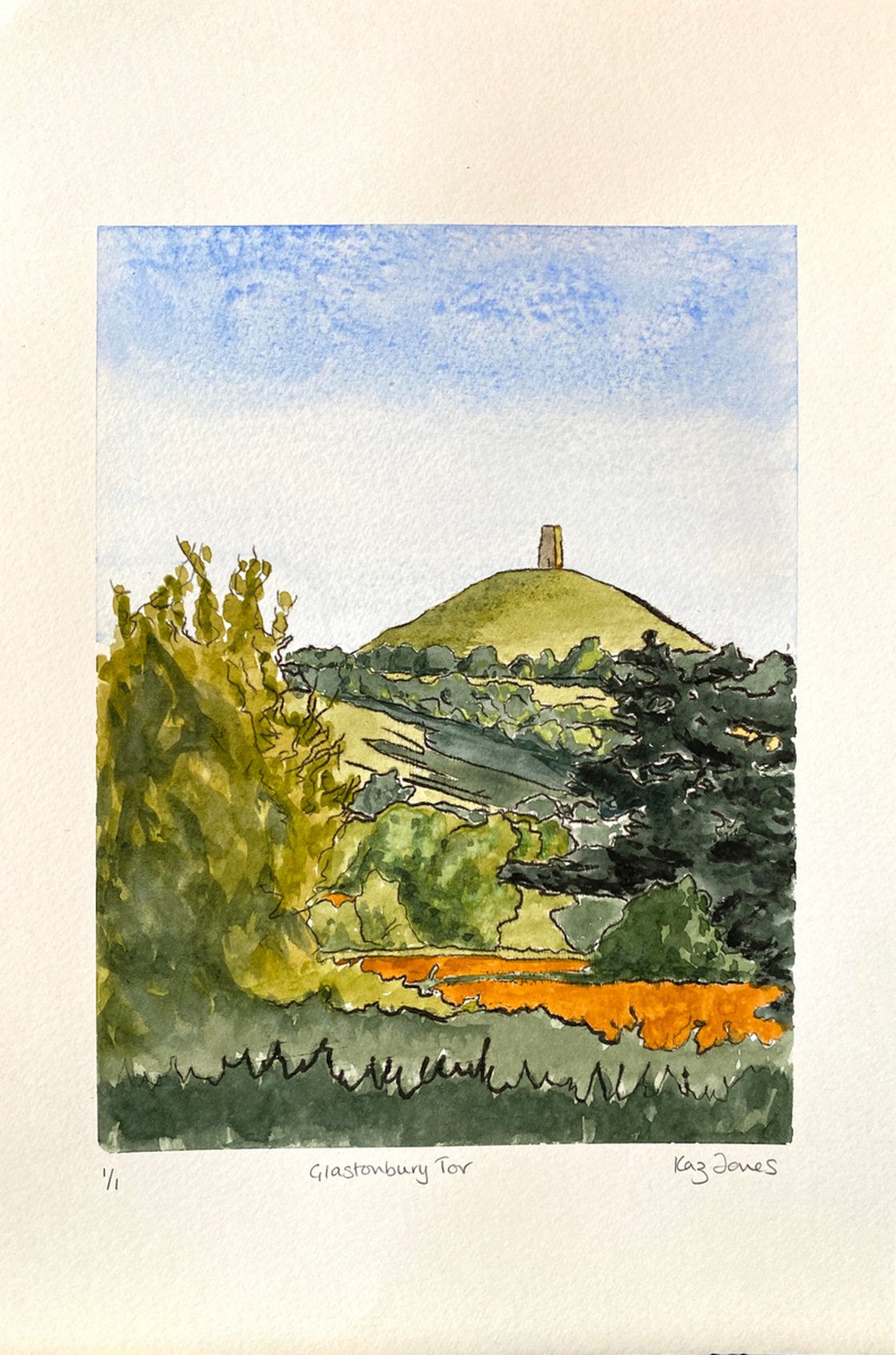This detailed watercolor painting, entitled "Glastonbury Tor," beautifully captures the serene landscape of a hillside. Created by the artist Kaz Jones in a sketchbook format, the painting is labeled "1/1" in the bottom left corner. Predominantly depicted in lush greens and vivid oranges, the foreground features a mix of olive-colored bushes on the left and medium to dark green trees on the right. Between these trees lies a field of orange, suggesting autumnal grasses. The central feature of the composition is a grassy hilltop crowned by a tan-colored monument or obelisk. Above this striking landmark, the sky transitions from a bright blue at the top to a very light, almost white, near the horizon. Enhanced by delicate pen outlines, this piece is framed by a white border and carries a personal note: "Painted by Kaz Jones" on the bottom right. Each element combines to create an evocative portrayal of the tranquil, scenic beauty of Glastonbury Tor.